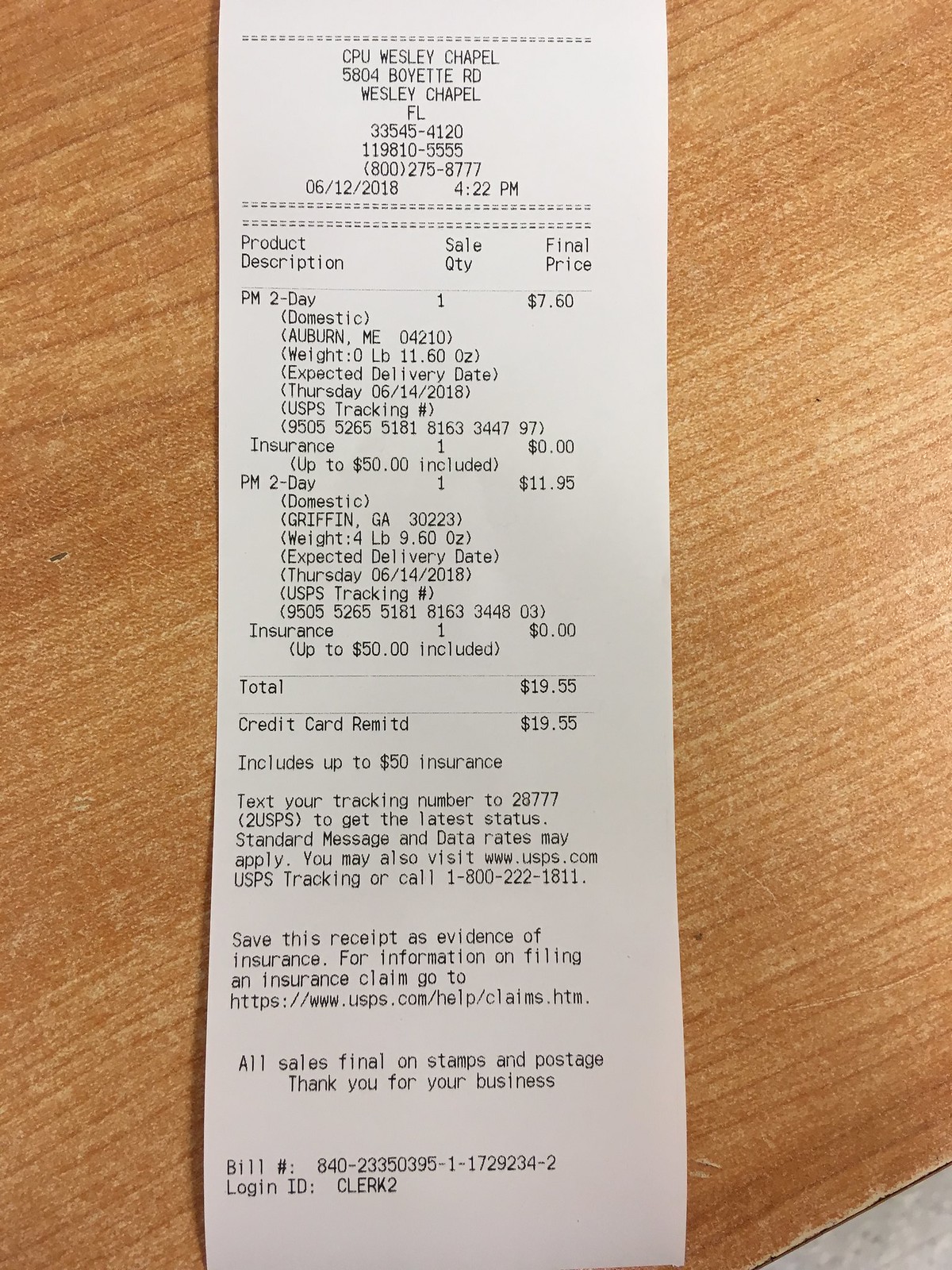This image depicts a detailed store receipt from a post office located in Wesley Chapel, Florida. The receipt outlines the purchase of shipping services, specifically two-day domestic mail, with each package costing $7.00 each. The expected delivery date for both packages is June 14, 2018. The receipt details include the USPS tracking number, confirming its authenticity as a post office receipt, and notes that $50 insurance coverage was included for each item. Additionally, it mentions that one of the packages is being sent to Griffin, Georgia, with the same arrival date of June 14, 2018, as the other item. Overall, the total cost of the transactions on this receipt amounts to $19.55.